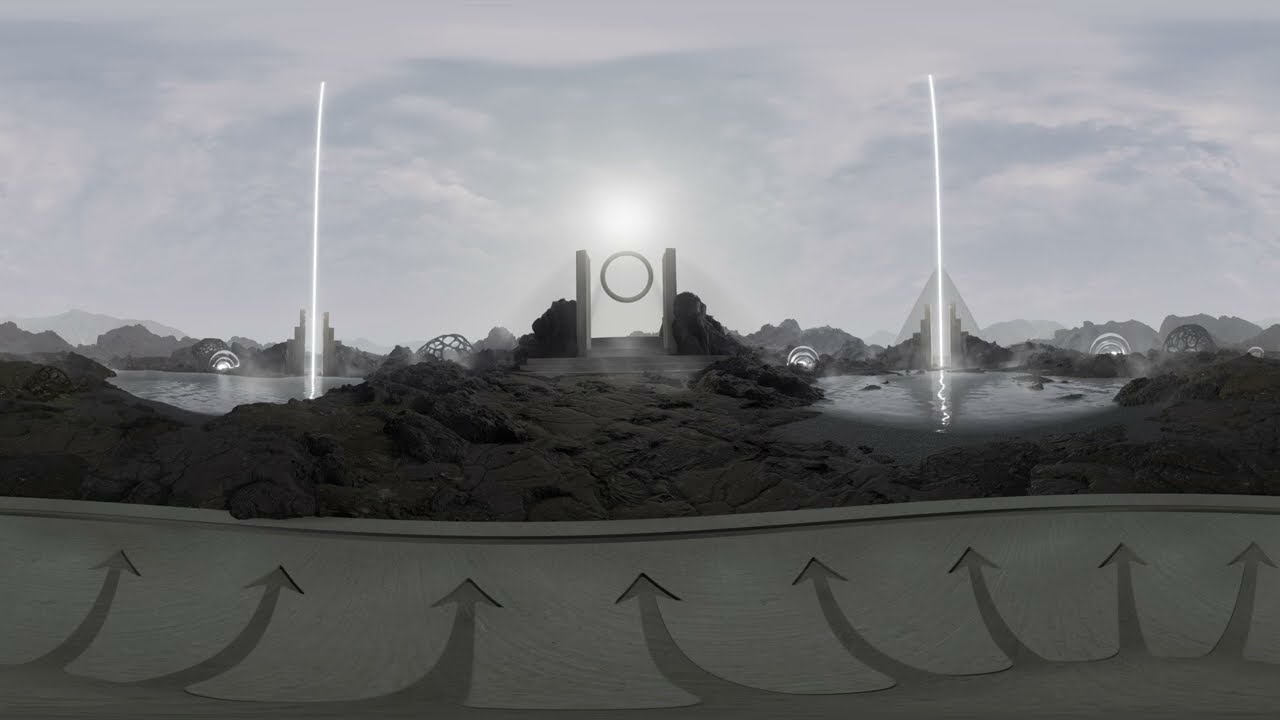A black and white image depicts a surreal, possibly computer-generated, scene with a blend of natural and futuristic elements. Central to the composition are two tall, parallel columns flanking a floating ring or circular emblem, which appears to be suspended mid-air between them. This emblem has a bright white center outlined by a darker gray border. The scene is divided into two sections, each featuring a body of water with rocky shores populated by scattered cylindrical structures and spherical orbs that seem partially submerged. 

Distinctly, there are two intense beams of light or electricity shooting down into each water area from above, resembling lightning bolts. In the foreground, a platform with arrows guides the viewer’s eye towards the central floating ring. Surrounding this platform are dense bushes that, despite the monochromatic palette, hint at verdant greenery. On the far left and right of the image, the beams of light glow against a backdrop that includes triangle or pyramid-like shapes, adding to the uncanny and fantastical atmosphere of the image.